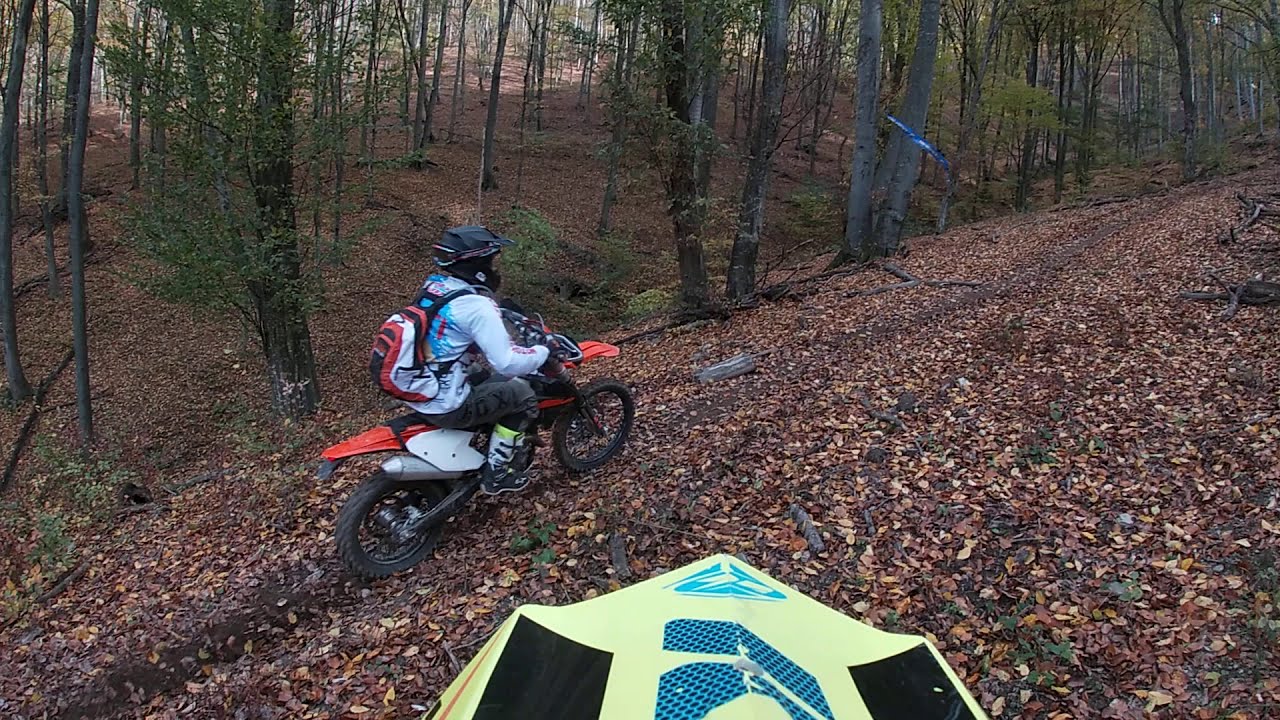In this image, we see a vibrant fall woodland scene featuring a dirt path covered in a rich tapestry of brown, orange, and yellow leaves. Winding uphill, the path is flanked by trees with green leaves, their skinny trunks reaching toward the sky. Prominently placed at the bottom center of the image is a piece of equipment, yellow with blue parts and some black sections on its sides. Dominating the scene is a man, dressed in a white shirt, black pants, and a black helmet, riding a red and white dirt bike with black tires. He carries a red and white backpack on his back as he navigates the leafy, muddy path that climbs toward the right. The scene suggests the perspective from atop another helmet, which is lemon in color with blue decorations. Additional blue and unidentified objects are scattered throughout the background, adding to the complexity of the forested landscape.